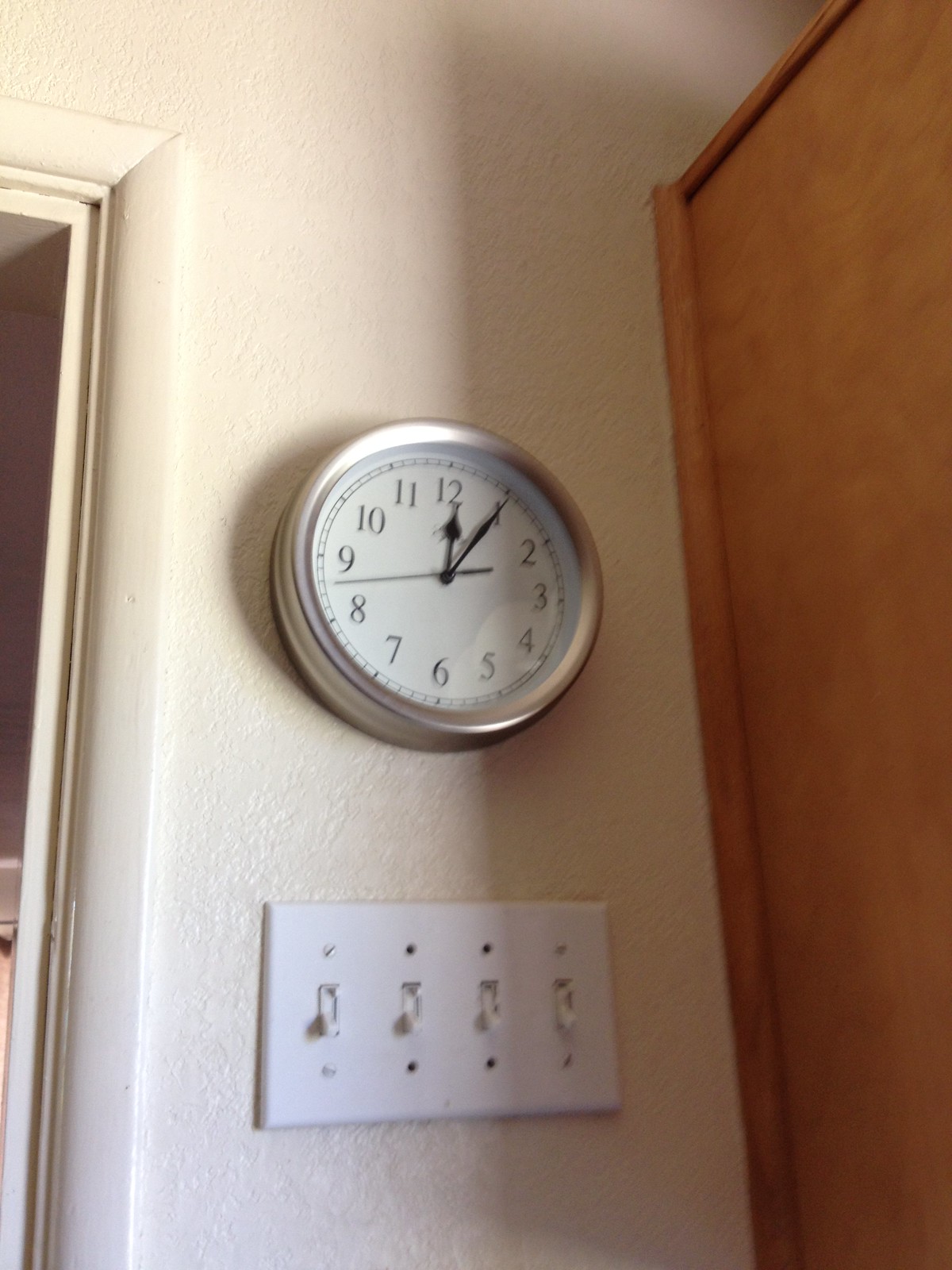This photograph, taken during the daytime, captures a detailed scene of a wall clock mounted on a narrow section of white, textured wall between two doorways. To the left, there's a white-painted doorframe, partially revealing a room through a hallway. To the right, a built-in wooden cabinet extends from the top of the doorframe down to the edge of the picture, showcasing light blonde wood. The wall clock, slightly narrower than the adjacent light switch panel, features a silver case with a thick base. The clock face is white, adorned with large black numbers, a prominent black second hand, a slender black minute hand with a spade-shaped pointer, and a sleek hour hand. The time displayed is 12:05. Beneath the clock is a rectangular light switch panel with four switches, surrounded by eight screws—four black screws centered above and below each switch, and four outer screws that are painted over. The setup casts shadows over part of the clock and the light switch panel, adding to the composition of the image.